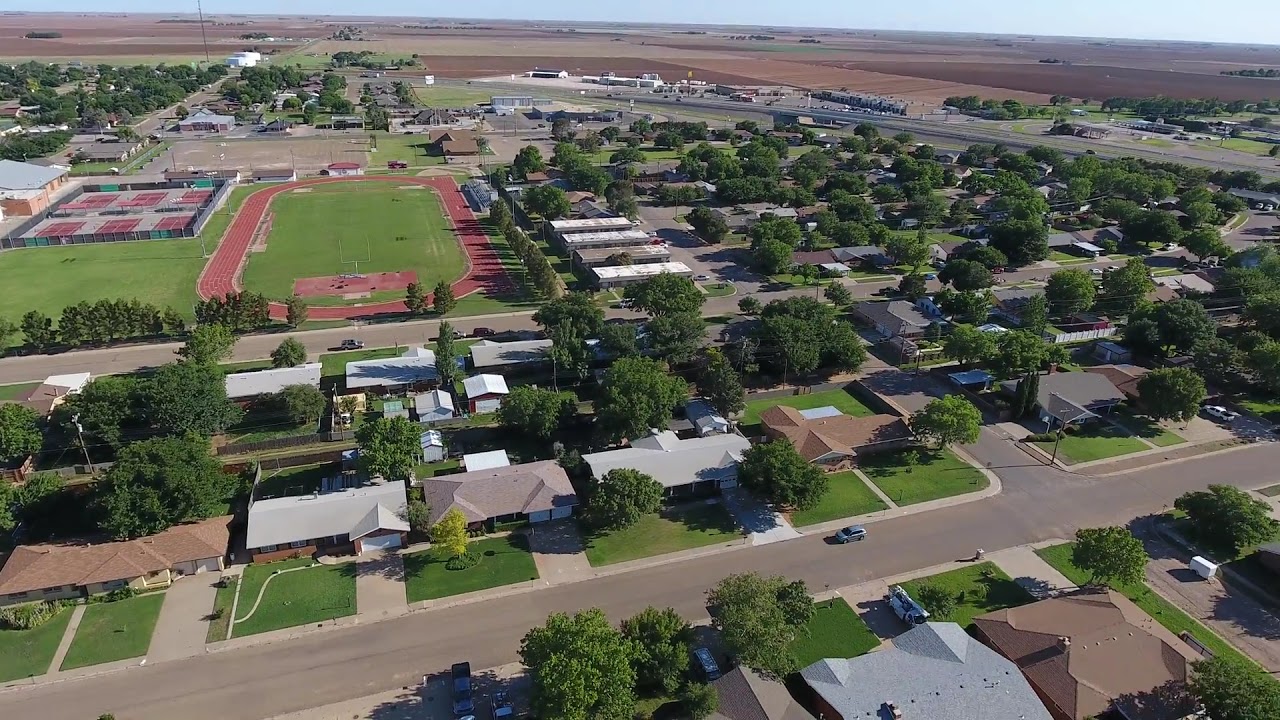This overhead photograph, taken by a drone or helicopter, intricately captures a neatly designed suburban neighborhood. In the lower foreground, rows of uniform, one-story ranch-style homes are visible, each situated on lush green lawns with driveways extending to the well-defined streets. A solitary vehicle traverses a neighborhood street, underscoring the quiet residential ambiance. The meticulously manicured lawns and big bushy trees further enhance the suburb's orderly appearance.

Towards the middle of the image, more houses and streets form a structured grid, with the rooftops of several homes prominently displayed. The upper portion of the image reveals a broader landscape, including open brown fields and a concrete tarmac road.

In the upper left corner, there's a detailed view of an athletic field belonging to the local school. This field features a red rubberized track encircling a green infield, with adjacent tennis courts and a paved parking lot beyond them. The thin ribbon of blue sky on the horizon adds a serene backdrop to this quintessential suburban scene.